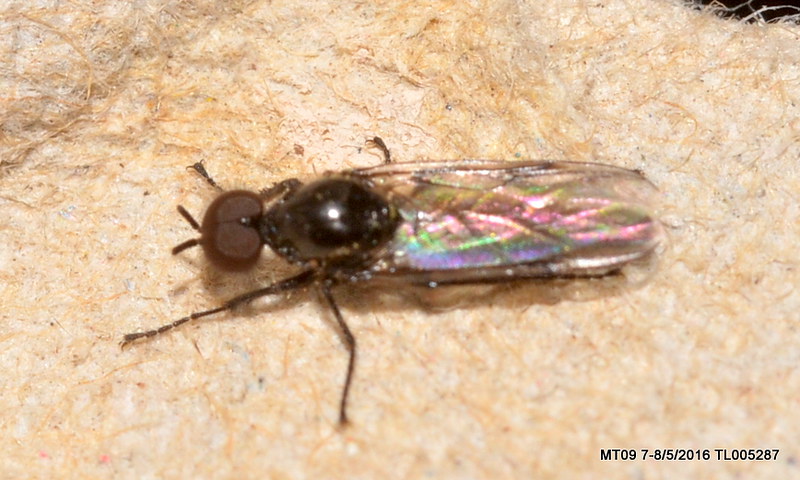This detailed close-up photograph captures an insect that resembles a fly, positioned centrally on an orange, fibrous material that could be cloth or possibly carpet. The insect features a black head with prominent, large eyes, accompanied by two antennas. Its body, which appears to have a hard shell, is predominantly black, while its wings are somewhat transparent and shiny, extending from its back. The legs, thin and black, are spread out across the surface. The insect's pose and appearance suggest it may not be alive. At the bottom of the image, there are some identifying numbers and text that read, "NTO97-852016 TL005287."